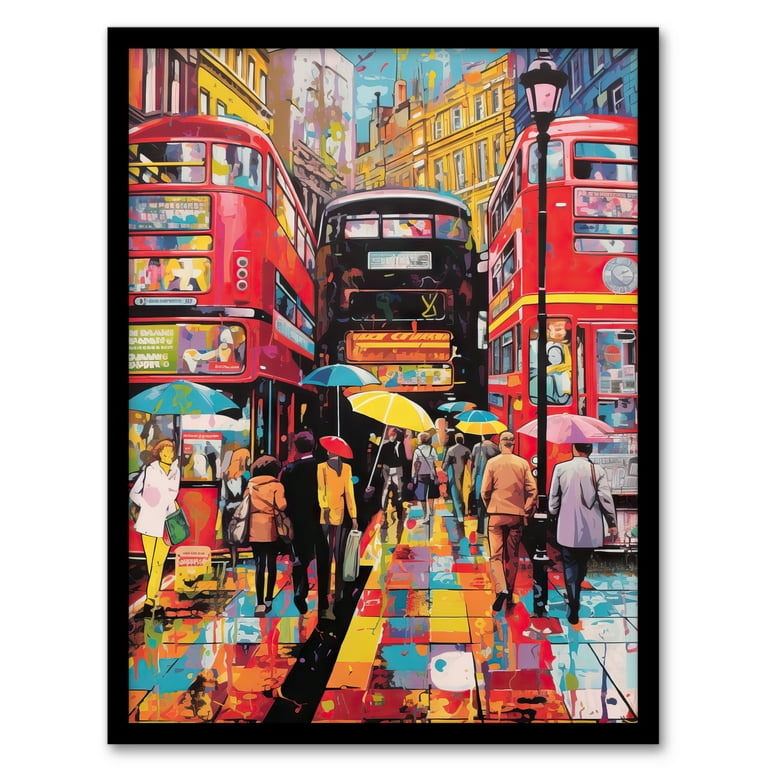This vibrant and colorful painting, framed in black, depicts a bustling street scene reminiscent of London, with its distinctive double-decker buses and a plethora of pedestrians. The animated, cartoon-like artwork features three double-decker buses prominently in the center: two red buses on either side of a black bus. Surrounding the buses are numerous people walking, many holding umbrellas in shades of yellow, blue, and pink, adding to the lively atmosphere.

Above the street scene, the background showcases a series of tall buildings with numerous windows, painted in hues of yellow, white, and dark blue. The sky is a splatter of blue, contributing to the dynamic, impressionistic style of the piece.

The ground or sidewalk at the bottom of the painting is an eclectic mix of bright, swirling tiles in various colors such as blue, yellow, orange, red, purple, and turquoise, giving the impression of a painted mosaic or the remnants of a painter’s palette. Among the details, a large black streetlamp stands out, adding an element of structure to the whimsical, splattered aesthetic of the scene. The overall impression is one of vivid motion and color, capturing the lively essence of a rainy day in a bustling city.